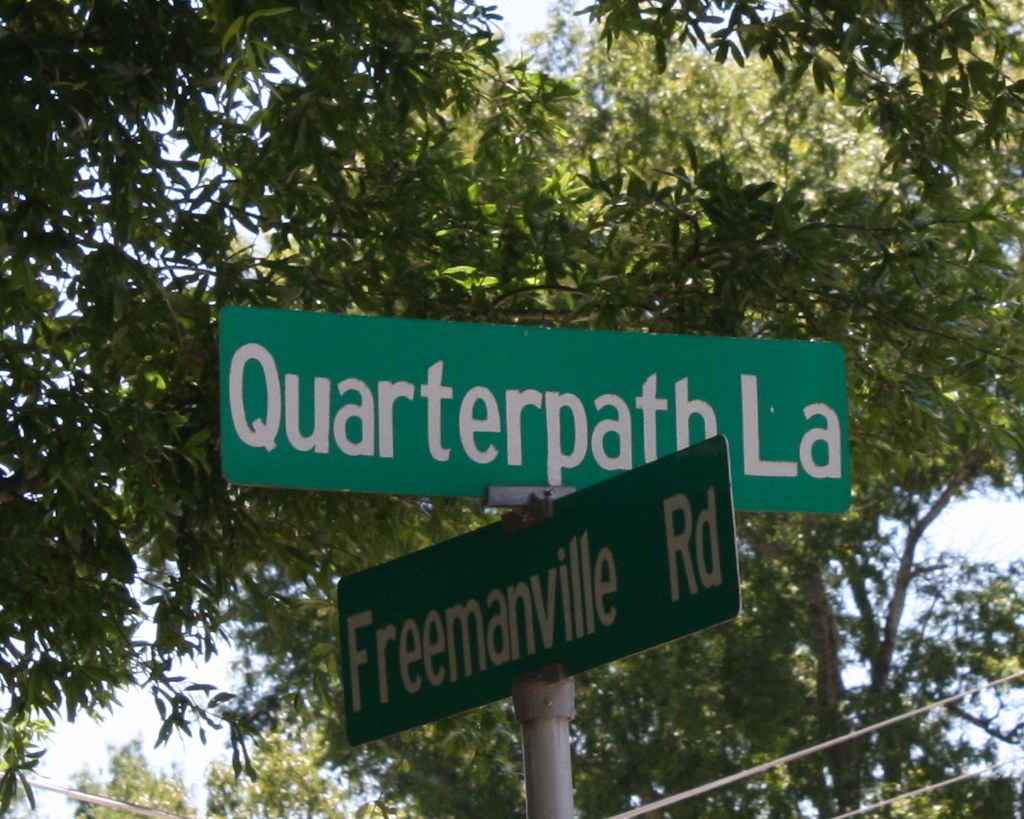This image captures a street corner, viewed from below with a focus on the intersection of two street signs. The metal pole holds two perpendicular signs: the top sign oriented horizontally reads "Quarter Path LA," while the bottom sign, vertically aligned, reads "Freemanville Road." Behind the street signs, a tree with lush green leaves creates a shadowy backdrop. The background features a clear blue sky, interspersed with power lines that either originate from or descend towards a nearby utility pole, adding an element of urban infrastructure to the outdoor scene.